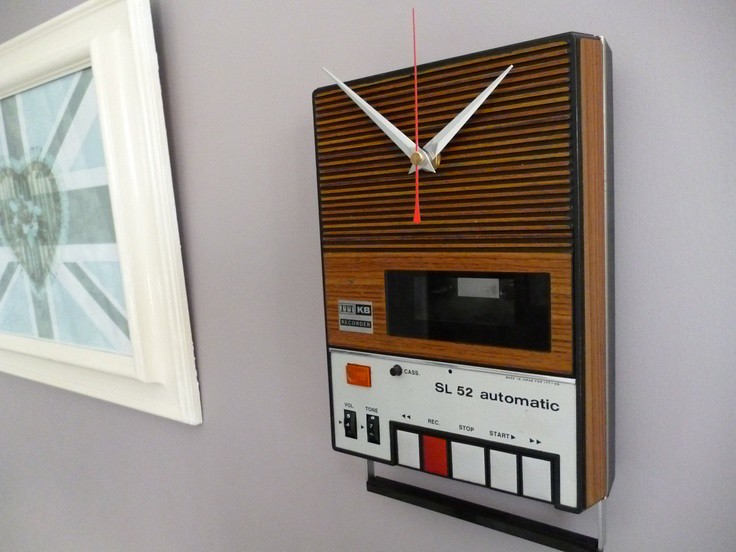This detailed photograph captures a wall-mounted clock that also functions as an answering machine, set against a light purple wall. Positioned directly behind the clock is a white-framed artwork featuring a heart and some vertical bars, rendered in shades of blue, gray, and white. The clock, constructed with stylized elements, has silver hands: the second hand points straight up, while the hour and minute hands indicate the time as approximately 1:53. Below the clock face is a cassette tape compartment, which has "KB" inscribed in a silver box on its left side. The lower segment of the device is white and features several control buttons—back, record (in red), stop, and forward—all in white, and labeled "SL-52 automatic." Additionally, there are volume and tone dials located on the left side of the answering machine. The overall design of the clock includes a plastic wood-grain finish in brown with horizontal darker streaks, accentuated by a black frame.